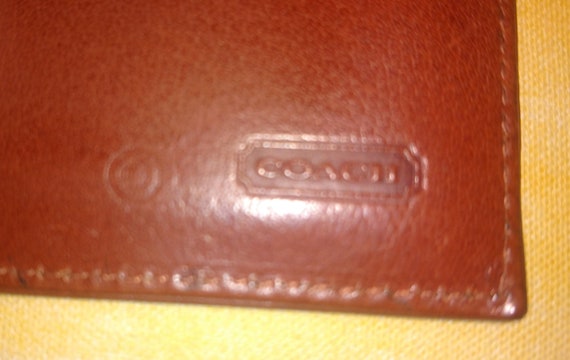The image is a close-up, slightly blurry photograph of the bottom right corner of a reddish-brown Coach leather item, likely a wallet. This rectangular picture, approximately four or five inches wide and three inches tall, presents the embossed Coach logo in the lower right corner, highlighted subtly by light reflection. Prominent stitching is visible along the edges, securing the leather to a thick, golden-yellow fabric, which covers the remaining portion of the image. This fabric, possibly a synthetic nylon, suggests a durable weave. The item is positioned against a yellow, textured background, possibly a tablecloth, providing a contrasting backdrop to the leather.